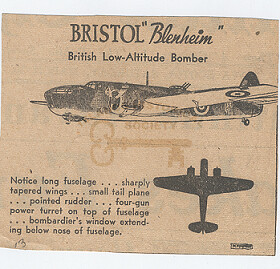This very old pamphlet, resembling a browned newspaper clipping with a tan background, prominently features the Bristol Blenheim British low-altitude bomber. At the top, black text labels the pamphlet with the aircraft's name. In the center, there is a striking gold key with the word "Society" in gold above it, though another, unreadable word precedes it. The centerpiece of the pamphlet is an illustration of the plane: its left side in black, the wing in white with a black bullseye underneath, and another bullseye on the plane's side. In the bottom right, a silhouette of the plane from an underside perspective is shown. Descriptive text in the bottom left highlights features like the long fuselage, sharply tapered wings, small tail plane, pointed rudder, four-gun power turret on top of the fuselage, and a bombardier's window extending below the nose of the fuselage.